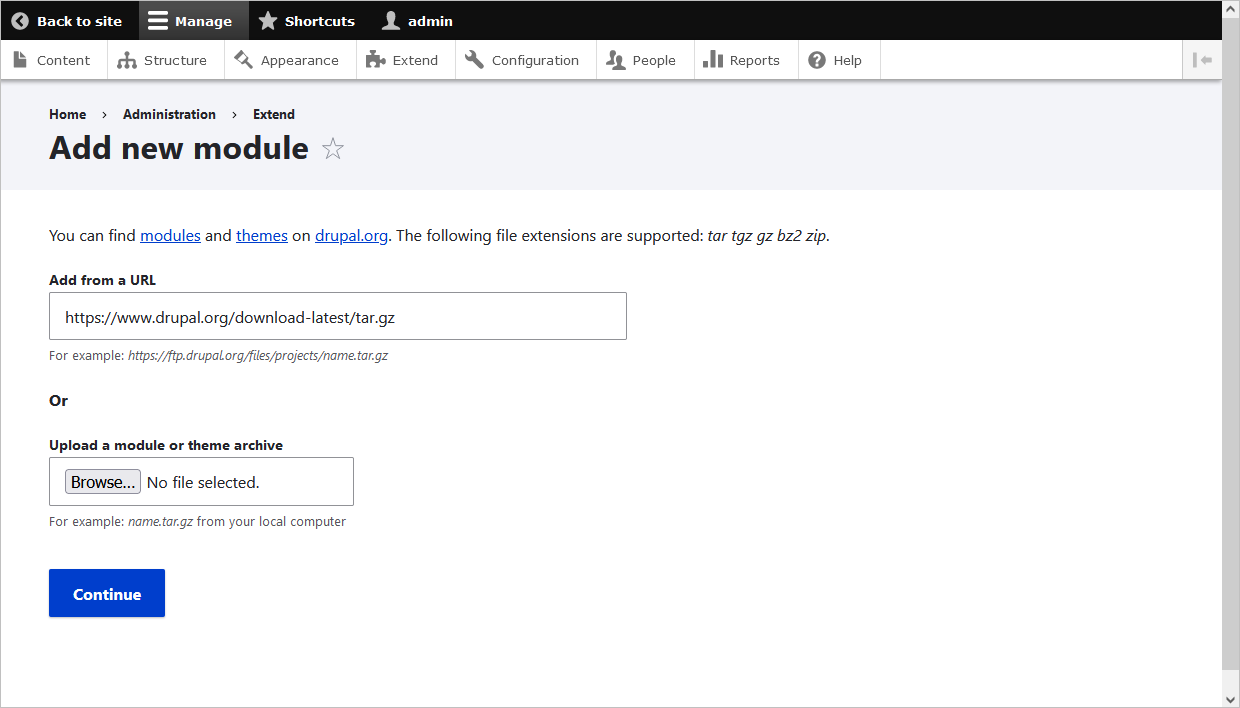This is a computer screenshot featuring a content management interface. A black horizontal bar spans the top of the screen. In the upper left corner of this bar, there is a gray circle containing a left-pointing black arrow. To the right of the circle, the words "Back to site" are written in white. Further right, three horizontal white lines are labeled "Manage". Proceeding further, a gray star icon labeled "Shortcuts" and then a head icon with the label "Admin" are visible.

Below this, a menu bar with a gray background runs across the width of the screen. Each menu item has an icon to its left and includes: Content, Structure, Appearance, Extend, Configuration, People, Reports, and Help. On the far right, a small gray square contains a vertical line and a dash on its right side.

Underneath these elements, another gray horizontal bar appears. In the top-left corner of this bar, "Home" is written in small bold black letters. Following it is a right-pointing arrow (sideways V) beside the label "Administration", and another arrow beside "Extend". Below this line, "Add New Module" is prominently displayed in bold larger black letters, accompanied by a gray star outline to its right.

The background below this header turns white. The phrase "You can find modules" appears, with "modules" in blue and underlined, then "and themes" in blue and underlined, followed by "on drupal.org" in blue and underlined. In black text, the sentence continues, "The following file extensions are supported for," followed by a list of supported file types.

Further down, in small bold black letters, "Add from URL" precedes a textbox containing a website address. Below this section are about three lines of text leading to the bolded word "or" and another textbox labeled "Upload a module or theme archive" with a "Browse" button inside it. Finally, approximately four lines below, a blue "Continue" button is present.